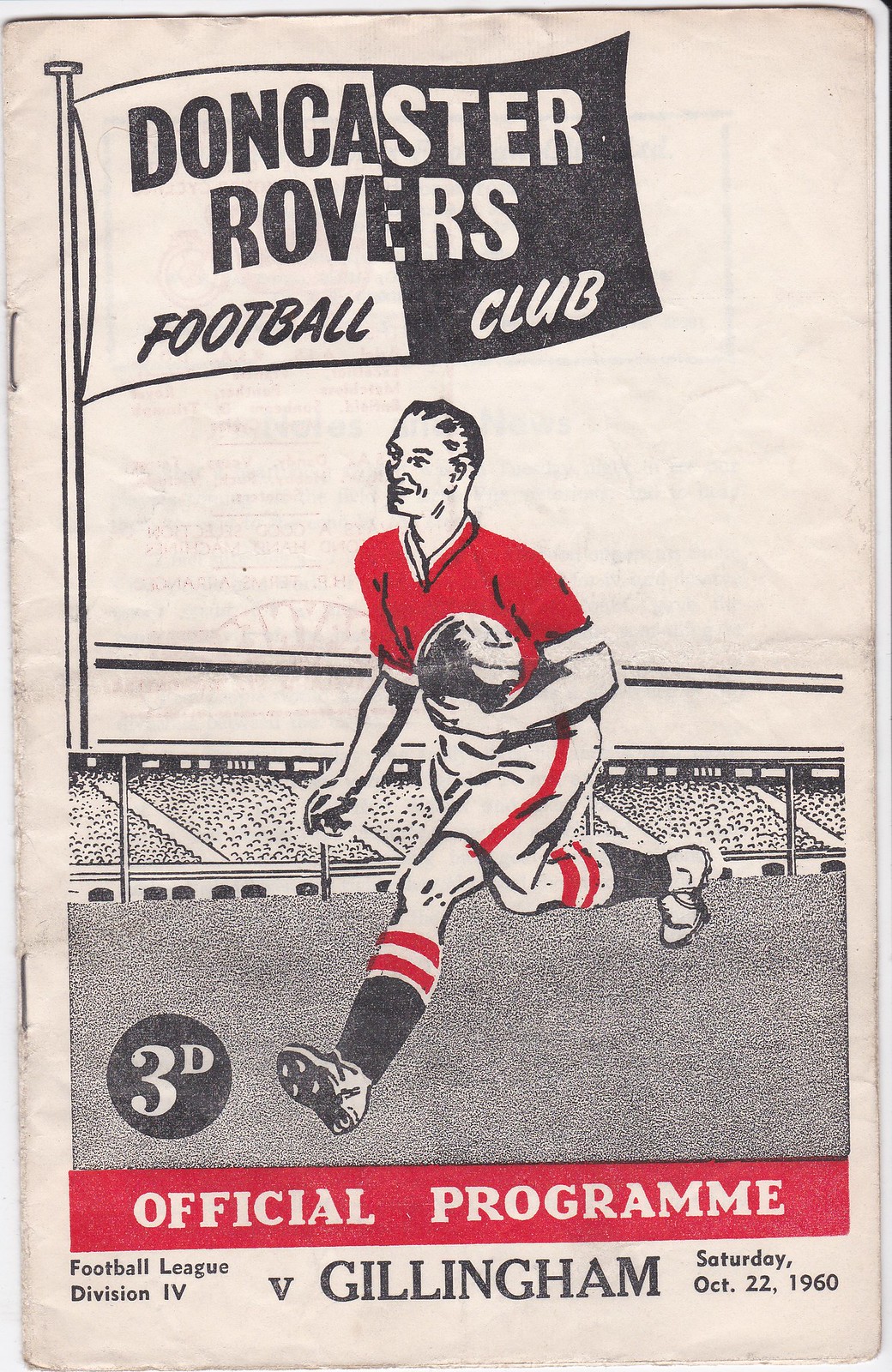This image is an official program cover for the Doncaster Rovers Football Club's match against Gillingham, held on Saturday, October 22, 1960, in Football League Division 4. The cover, which looks remarkably aged and is printed on faded beige paper, features a central illustration of a football player in action. The player is dressed in a red jersey, white shorts with red stripes, red-striped socks, and cleats. He is depicted running and holding a soccer ball in his left arm. The background includes a stylized drawing of a stadium, though the crowd is indistinct. A flag above the player bears the name "Doncaster Rovers Football Club" in alternating black and white lettering. A prominent red bar at the bottom with white letters indicates "Official Programme," and beneath this, in black text, it officially states "Football League Division IV vs Gillingham, Saturday, October 22, 1960." The overall design and elements give the cover an old-fashioned appearance, indicative of its 63-year-old vintage.